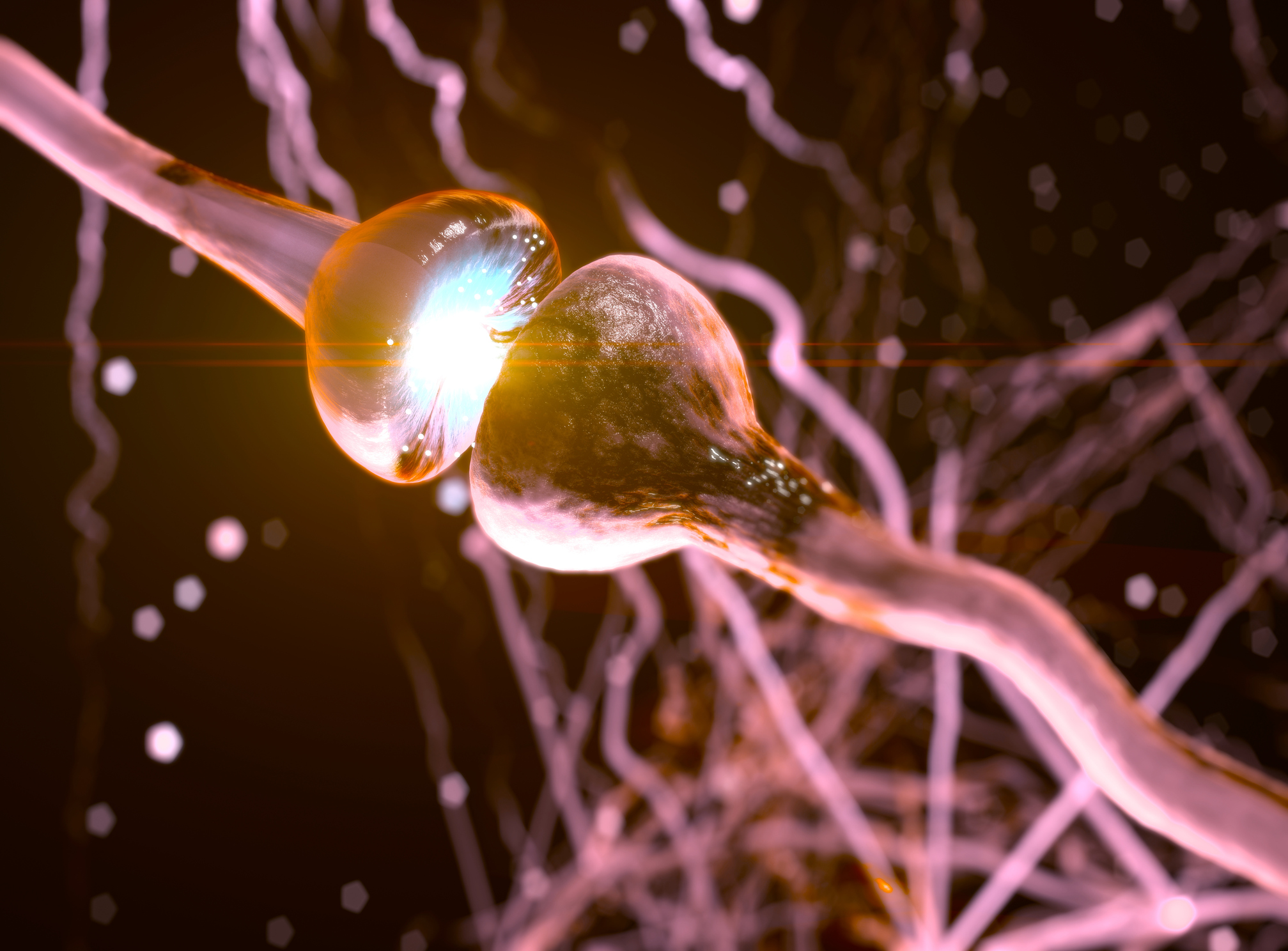This image appears to capture a surreal, close-up scene resembling either an alien-like realm or a microscopic environment, filled with vivid, otherworldly details. The focal point is two tube-shaped objects, each adorned with semi-circular, suction cup-like ends, subtly glowing with hues of yellow, blue, green, purple, and brown. One tube emerges from the top left, while the other approaches from the bottom left, nearly touching to form a complete circle. The left tube illuminates the scene with an eerie, multicolored light. The backdrop is a strikingly intricate network of vibrant purple and orange, intertwined like a distorted spiderweb, against a dark, blurred background dotted with small, glowing white and purple points. This intricate display might be an underwater scene or something microscopic, potentially an artistic creation, with every element meticulously painted or drawn to evoke a sense of mysterious, high-end art.